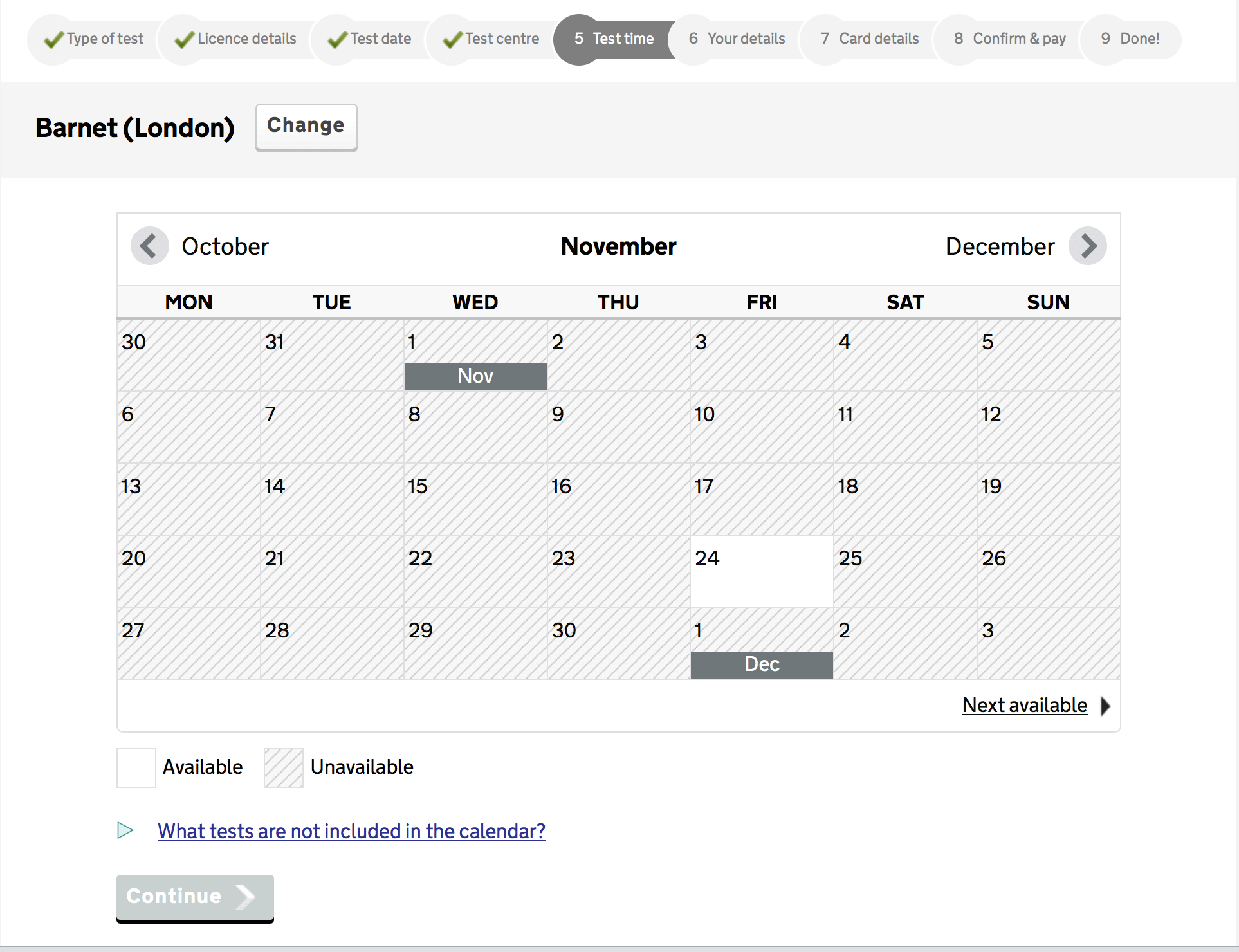This image depicts a website interface designed for scheduling a test. The webpage features a clean, white background and displays a progress checklist at the top, stretching from left to right. This checklist includes various steps necessary to complete the testing process. The initial tasks, marked with green checkmarks, indicate completed stages and include "Type of Test," "License Details," "Test Date," and "Test Center." The subsequent steps, which lack checkmarks, list “Test Time,” “Your Details,” “Card Details,” "Confirm and Pay," and "Done."

Just below this progress bar is a gray horizontal box displaying "Barnett London," with an adjacent button to change the location. Directly beneath this box is a calendar set to November, with navigation buttons allowing users to cycle between October and December. The calendar clearly marks dates ranging from the 1st to the 30th of November, along with the first three days of December.

A key below the calendar indicates date availability—white for available dates and gray for unavailable ones. The section also specifies which tests are not included in the calendar and concludes with a prominent "Continue" button.